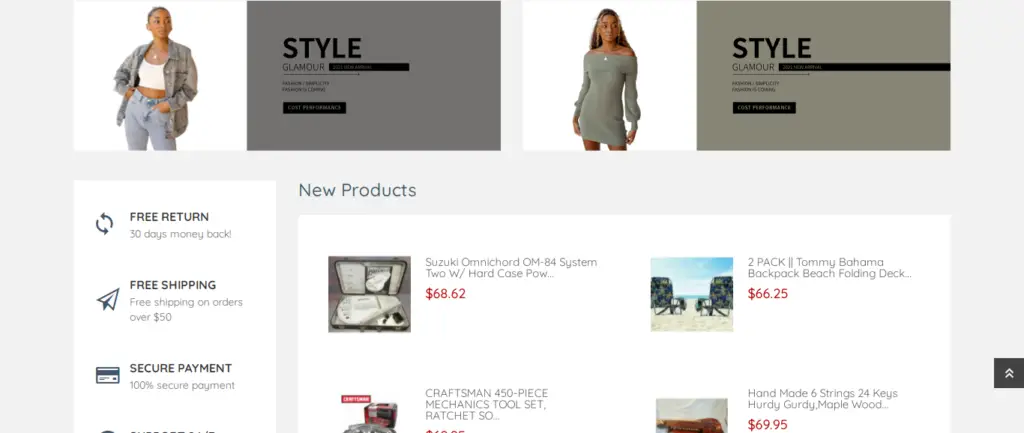The image appears to be a screenshot of an online shopping website on a computer screen. In the upper left corner, there is an image of a woman dressed in a gray jacket, white tank top, and blue jeans, with the word "Style" next to it. Some information adjacent to this has been obscured. Below this, another image showcases a woman wearing a gray dress, also labeled "Style," with additional blacked-out information beside it.

Underneath these sections is a white rectangle on the left that lists various customer benefits: "Free Returns, 30 Days Money Back, Free Shipping, Free Shipping on Orders Over $50, Secure Payment, 100% Secure Payment." 

To the right of this, another rectangle is labeled "New Products," listing items for sale. The items detailed include:
- "Suzuki Omni Cord System 2 with Hard Case, 6862."
- "2-pack of Tommy Bahama Backpack Beach Folding Deck Chairs, $66.25."
- "Craftsman 450-piece Mechanics Tool Set Ratchet." (The price is cut off).
- "Hand Mode 6-String 24T Hurley Gertie Maplewood, $69.95."